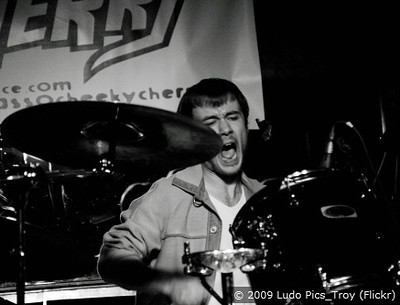The black and white photograph captures a man with a short haircut and dark, mid-length hair, energetically playing the drums and singing with his mouth wide open. He is dressed in a white t-shirt layered with an unbuttoned denim jacket. The top right corner of the picture includes part of a banner with large, partial letters, likely spelling "E R R Y," and smaller text below that reads "Cheeky Cherry." A prominent white flag featuring large lettering hangs behind him. Despite the very dark background, the scene is lit by a stage light that reflects off his drum kit, which includes visible cymbals and a drum. Only his upper body is visible in this small, detailed image, which is marked with the copyright notice "© 2009 Ludo Pics_Troy (Flickr)" in the bottom right corner.